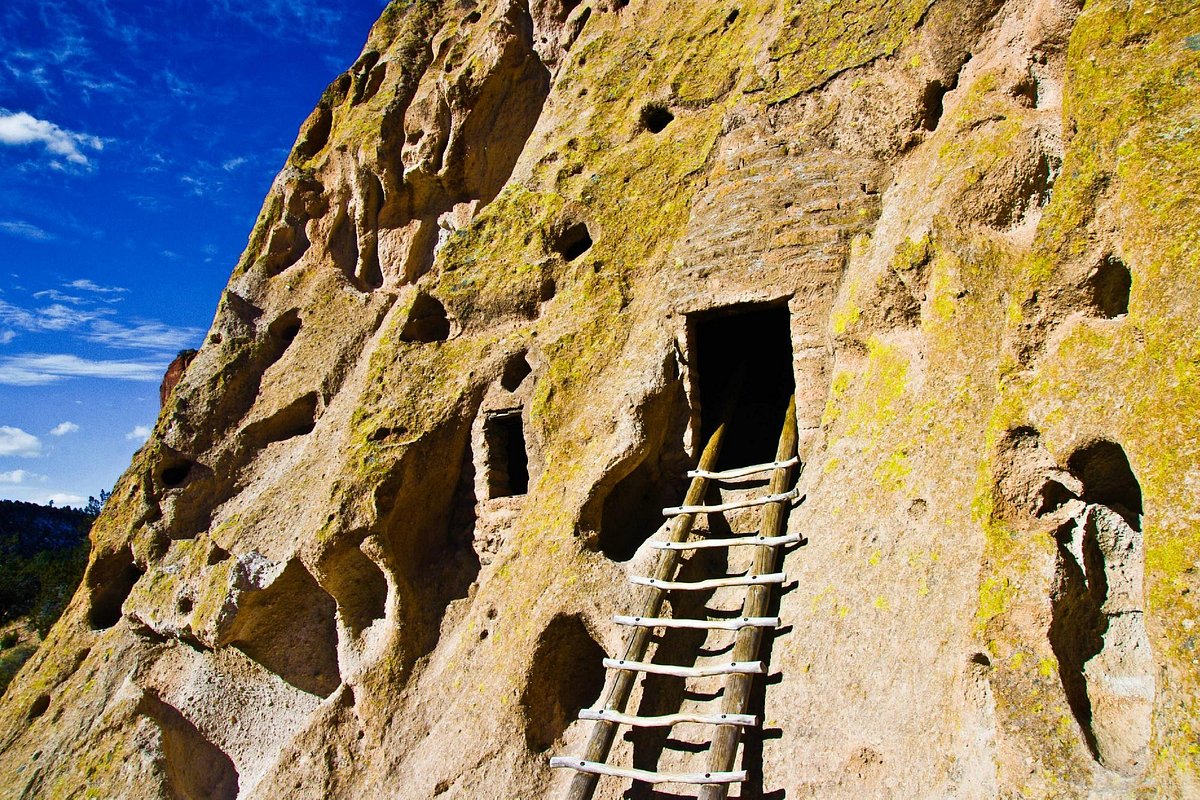The photograph, taken outdoors at Bandelier National Park, showcases a stony cliffside with rectangular doorways cut into it, indicating ancient cave dwellings. A rustic wooden ladder, constructed with sticks and rungs, leans against the cliff, providing access to one of the central doorways. The cliffside is partially covered in vibrant green moss, especially prominent on the right side and surrounding some of the openings. The sky in the background to the left is a deep, vibrant blue, adorned with scattered white clouds, adding a striking contrast to the earthy tones of the mountain and its man-made structures.